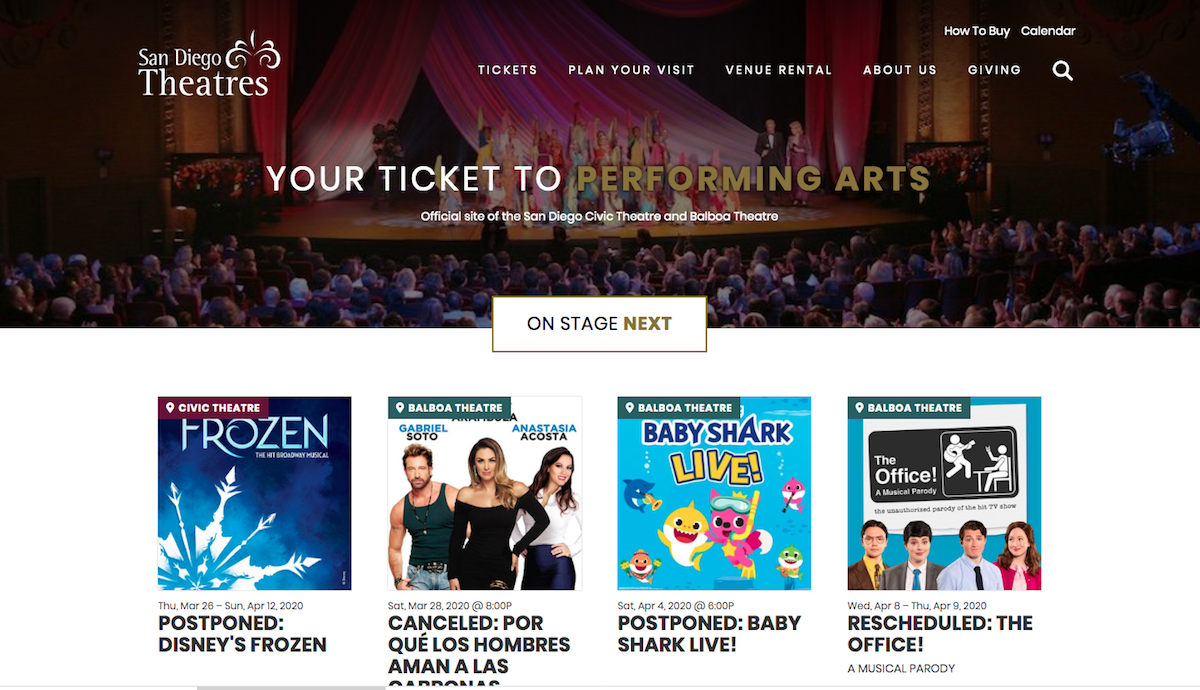This detailed caption describes a screenshot of a web page related to San Diego Theatres. 

---

**Caption:**

Screenshot of the official San Diego Theatres website. The page, cropped to exclude browser information and the bottom section, features a rich background photograph of a stage performance in a classic, old-style theatre filled with a large audience. The "San Diego Theatres" logo is prominently positioned in the top left corner. 

Running along the top is a navigation menu, which includes links for "Tickets," "Plan Your Visit," "Venue Rental," "About Us," and "Giving," alongside a search button. The main headline, "Your Ticket to Performing Arts," introduces the site’s purpose of selling tickets for the San Diego Civic Theatre and Balboa Theatre.

The section visible towards the bottom showcases four upcoming events with graphical images and event details beneath them. These events are: "Frozen," an event with a title in Spanish, "Baby Shark Live," and "The Office: A Musical Parody."